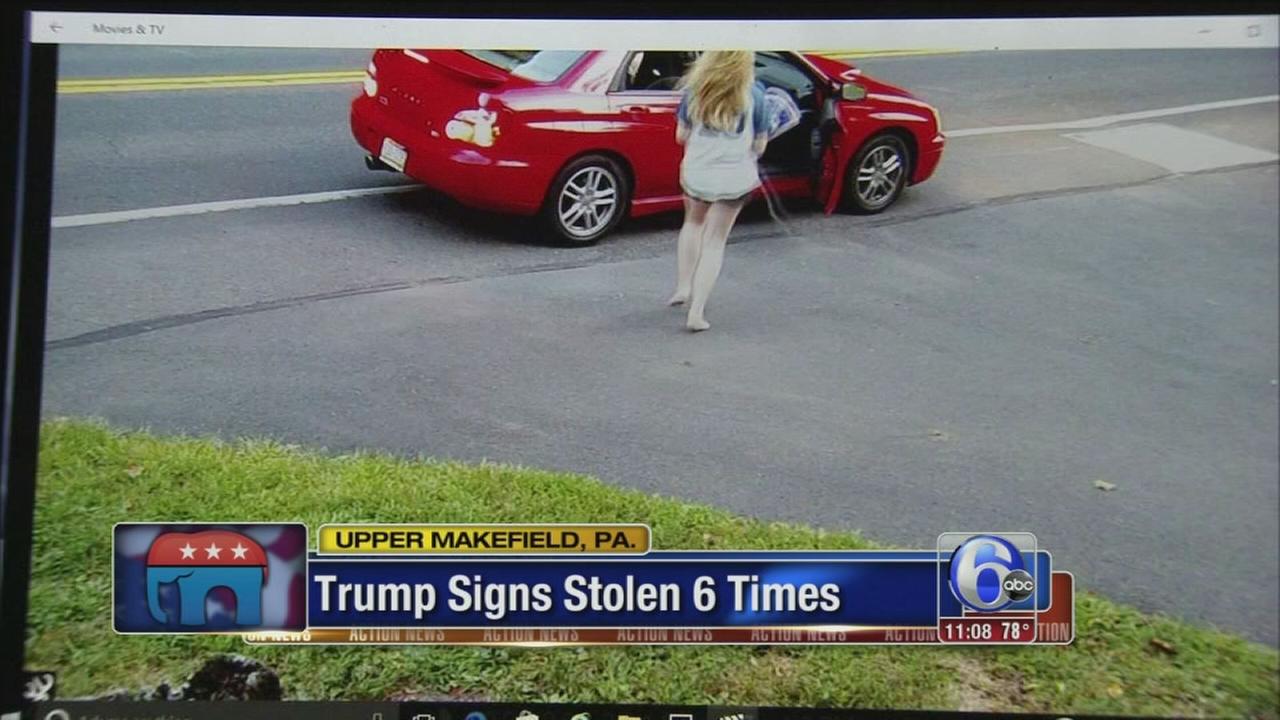The image appears to be a screenshot of a TV newscast, with a wide, horizontal black background framing the scene. At the top left corner of the screen, there's a light gray horizontal rectangle featuring the heading "Movies and TV." The central portion displays a young blonde woman with long hair walking towards a red car, possibly a Subaru Impreza, with its door open on a gray concrete road. The woman is wearing a blue and white t-shirt, shorts, and knee-high white socks, and she's holding something with a wire. Green grass lines the other side of the road. Overlaying this scene is a graphic with a red and blue elephant symbol adorned with three white stars, accompanied by the text "Upper Makefield, PA Trump sign stolen six times." The bottom right corner of the screen shows the Channel 6 ABC logo, the time 11:08, and a temperature reading of 78 degrees, along with the "Action News" label.